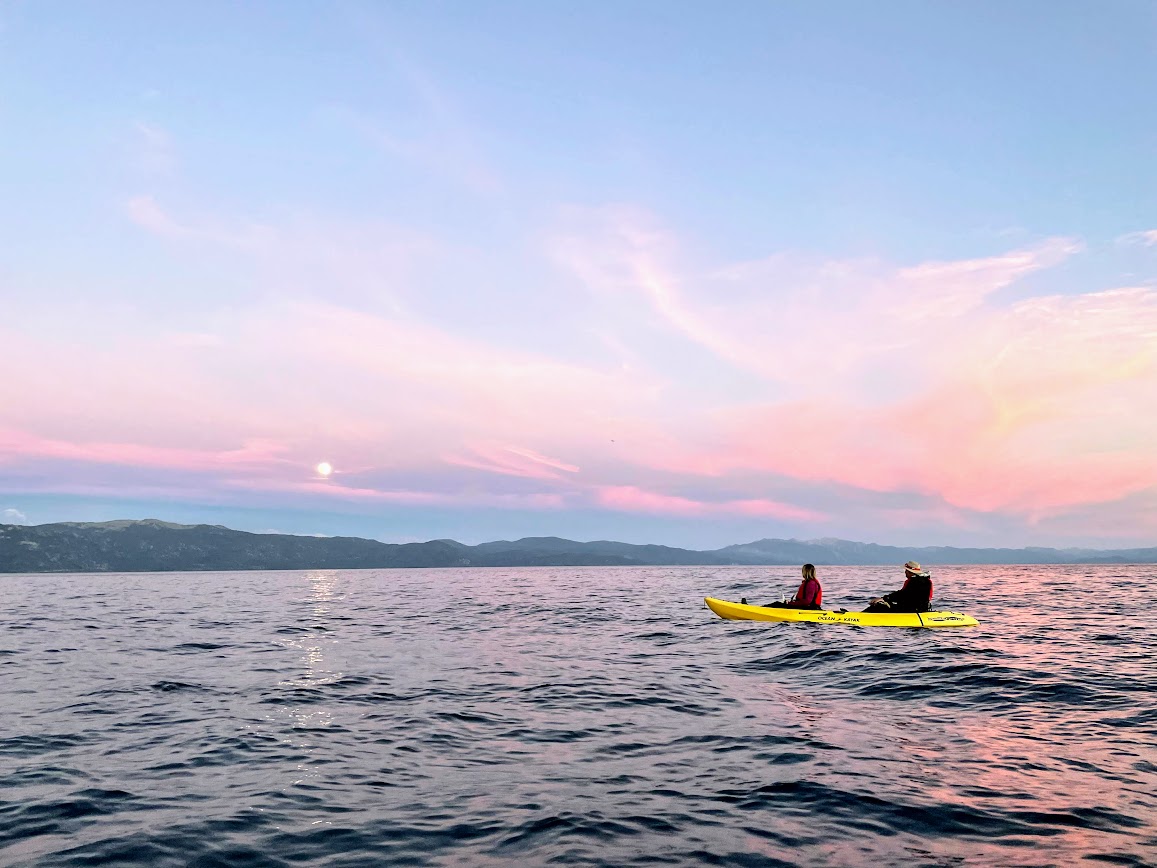In this outdoor scene captured near the water level, the sky is alive with a bubblegum blend of pinks, blues, and soft oranges, hinting at an ongoing sunset. The sun appears as a tiny dot low on the horizon, highlighting the tranquility of the moment. In the distance, dark, smooth hills line the horizon, adding depth to the serene setting. Dominating the foreground is a large body of water, slightly wavy, reflecting the multi-colored sky. To the right of the image, a yellow canoe or kayak with two individuals is moving towards the center. The person in the front, possibly a female with chin-length blondish-brown hair, wears a red shirt or jacket, while the individual in the back, likely a male in a dark coat and a beige brimmed hat, contributes to rowing. The picture is detailed, especially in the depiction of the water and the soft hues of the sky, creating a peaceful and reflective atmosphere.